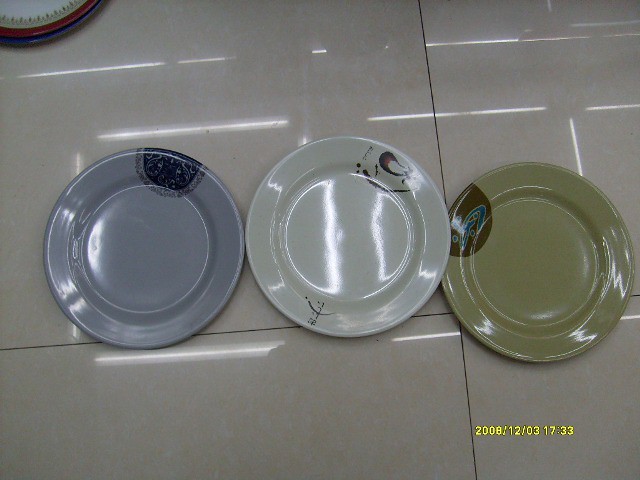This photograph captures an overhead view of three artisanal plates arranged on a highly reflective, glossy white tile floor. The light reflects off both the floor and the central plate, creating subtle streaks across the image. In the upper left corner, partially visible, is a stack of plates characterized by a variety of trims—blue, red, and white with a floral band. Centered and moving from left to right, the first plate is a striking gray with intricate blue etchings and a squiggly blue border. The next plate is white, adorned with brown etchings and green and brown designs, accompanied by a black mark. The final plate is olive green, featuring a distinct brown spot with blue accents. Notably, in the bottom right corner, a timestamp reads “2008/12/03 17:33.”